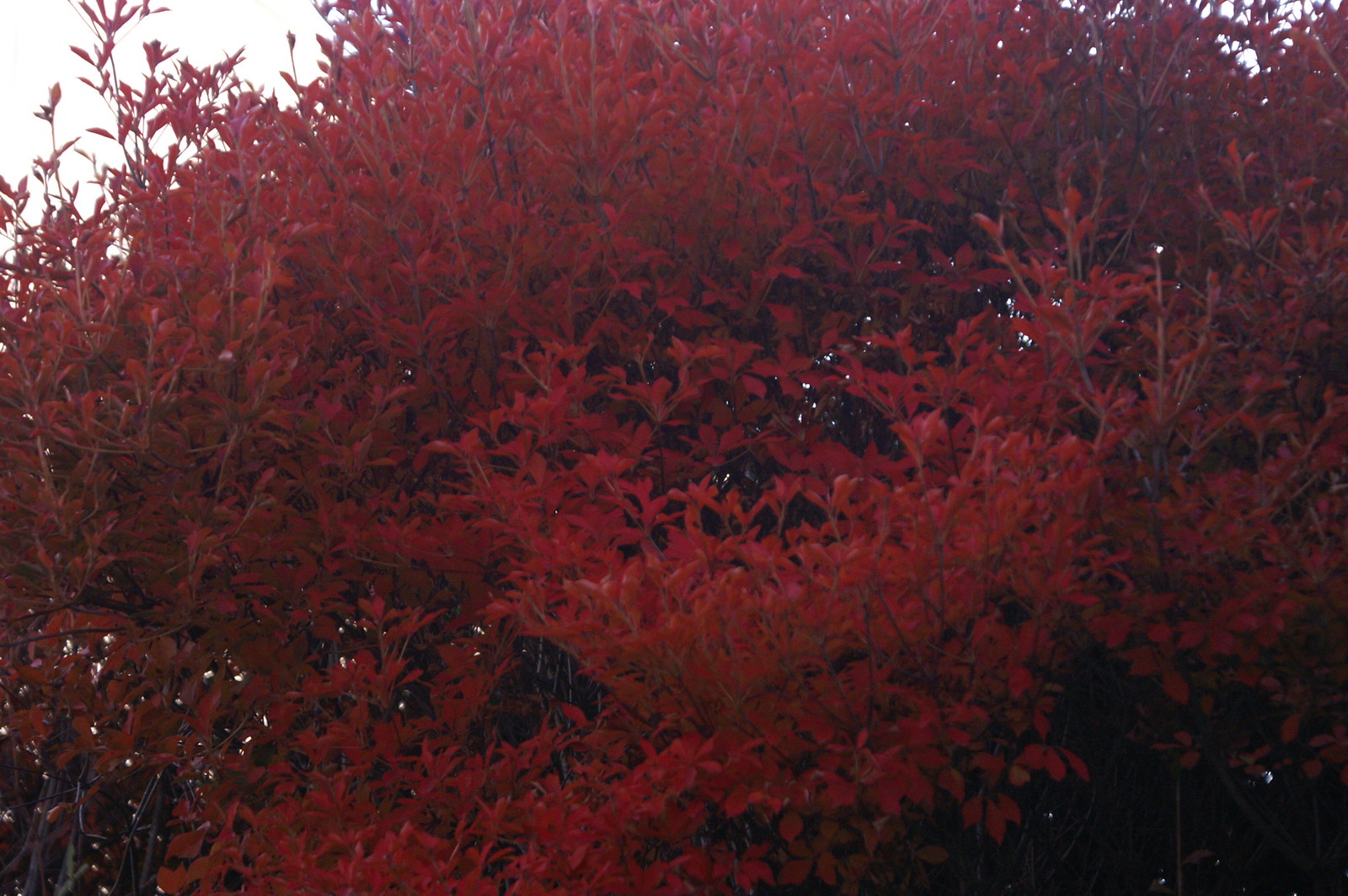The image features a close-up of a large and vibrant tree, possibly a Japanese red maple, showcasing its bright red leaves in full bloom, indicative of early spring. The lush foliage dominates the entire frame, with the red leaves creating a beautiful, flowery hue. Brown branches peek through the dense canopy, supporting the myriad of leaves. Tiny specks of light filter through small gaps, while the top of the image reveals a slightly larger area of sky, suggesting a sunny, perhaps mildly cloudy day. The setting appears to be an outdoor space, likely in a park or forest patch.